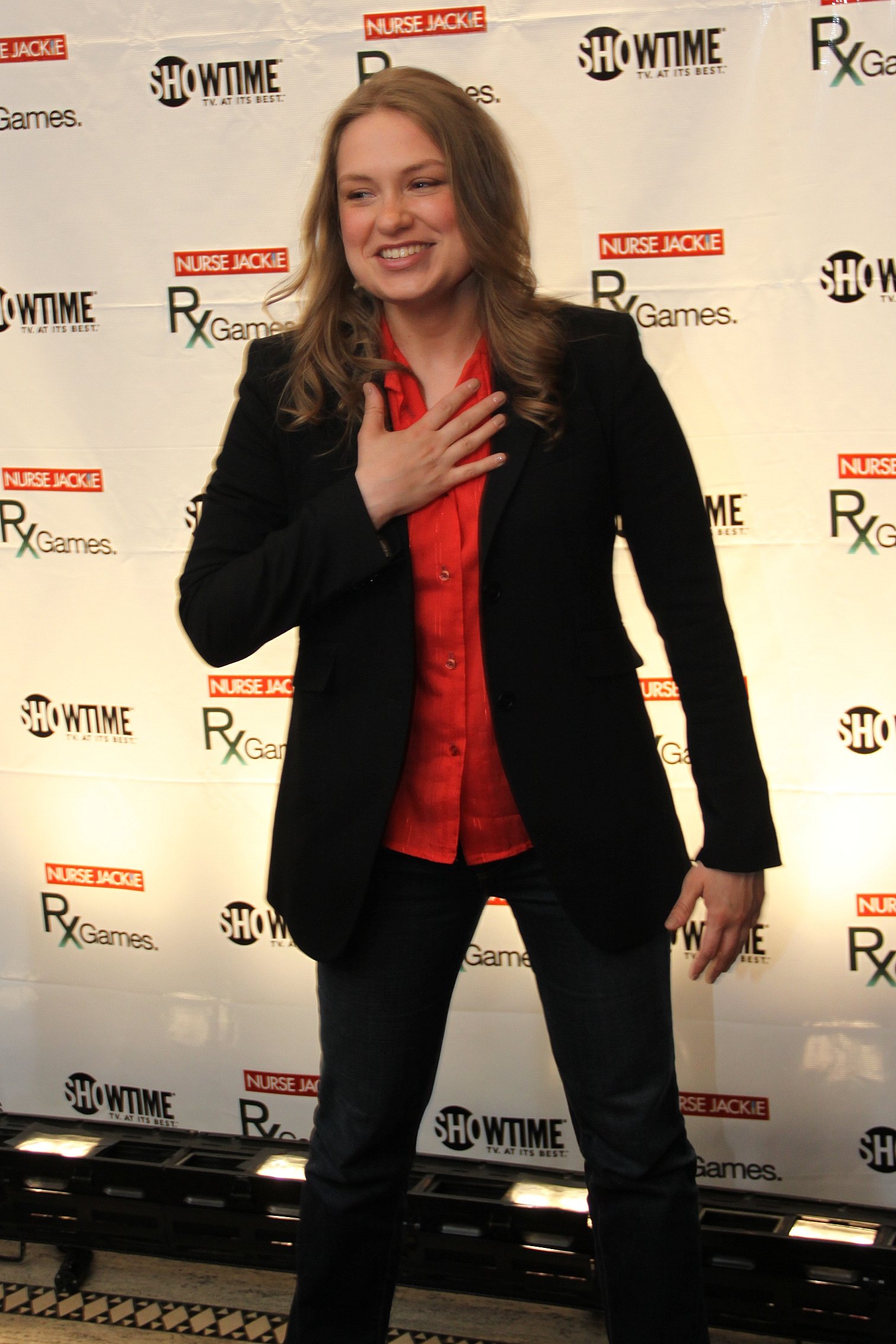This image is a color photograph of a smiling woman standing in front of a white background decorated with repeating logos for Showtime, Nurse Jackie, and RxGames. The backdrop features the Nurse Jackie logo in a red rectangle with white letters, and logos for RxGames and Showtime positioned around it. The woman, possibly an actress from the TV show Nurse Jackie, has long, light brown or dirty blonde wavy hair. She is dressed in a black sport coat over a red buttoned shirt, paired with black pants or dark blue denim jeans. Her right hand is touching her chest while her left arm rests at her side, and she appears to be striking a deliberate pose with a big smile on her face, looking pleased to be there.